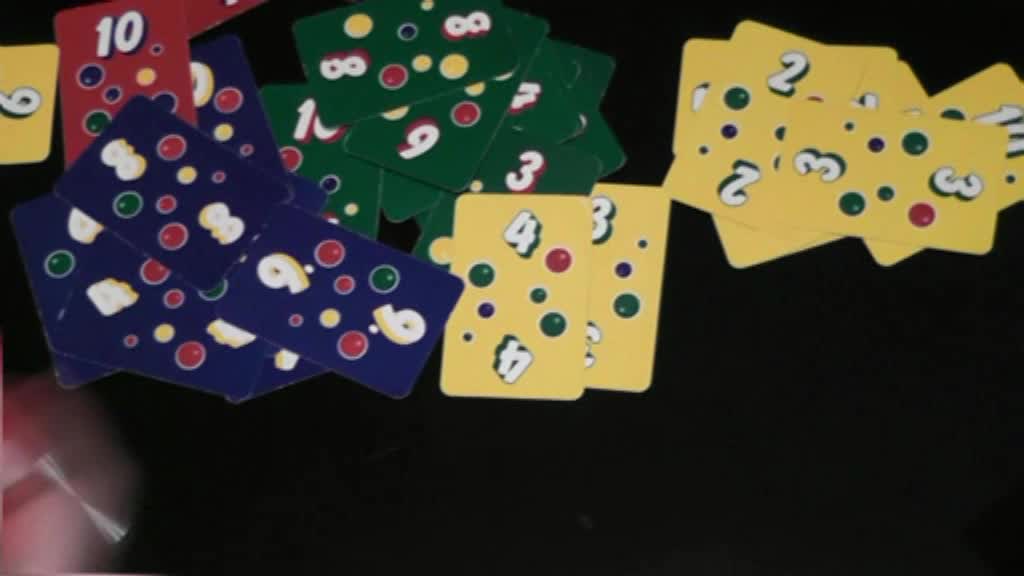A landscape photograph captures a card game spread out on a dark, black table. The table serves as the entire background, though the bottom left-hand corner appears quite blurry. A variety of colorful cards are clearly visible, arranged in different sections by their distinct hues.

In the upper left-hand corner, a solitary yellow card, marked with either a nine or a six, stands out. The rest of the yellow cards are grouped towards the center-right upper corner, displaying numbers such as four, three, two, three, and ten. Each yellow card features an array of dots: two large dark green dots, one large red dot, one medium blue dot, one medium green dot, and a small blue dot.

Two red cards, one marked with a ten, are located in the upper left corner. The upper center portion of the image displays a collection of green cards, totaling nine, with visible cards showing numbers eight, nine, three, and ten. One of the green cards, marked with either a nine or six, adds to the array.

On the left-hand side, a set of seven dark blue cards is arranged, revealing an eight, a blurry four, and a card that could potentially be either a nine or a six. The overall scene presents a vivid and organized array of cards, each differentiated by color and intricate details.